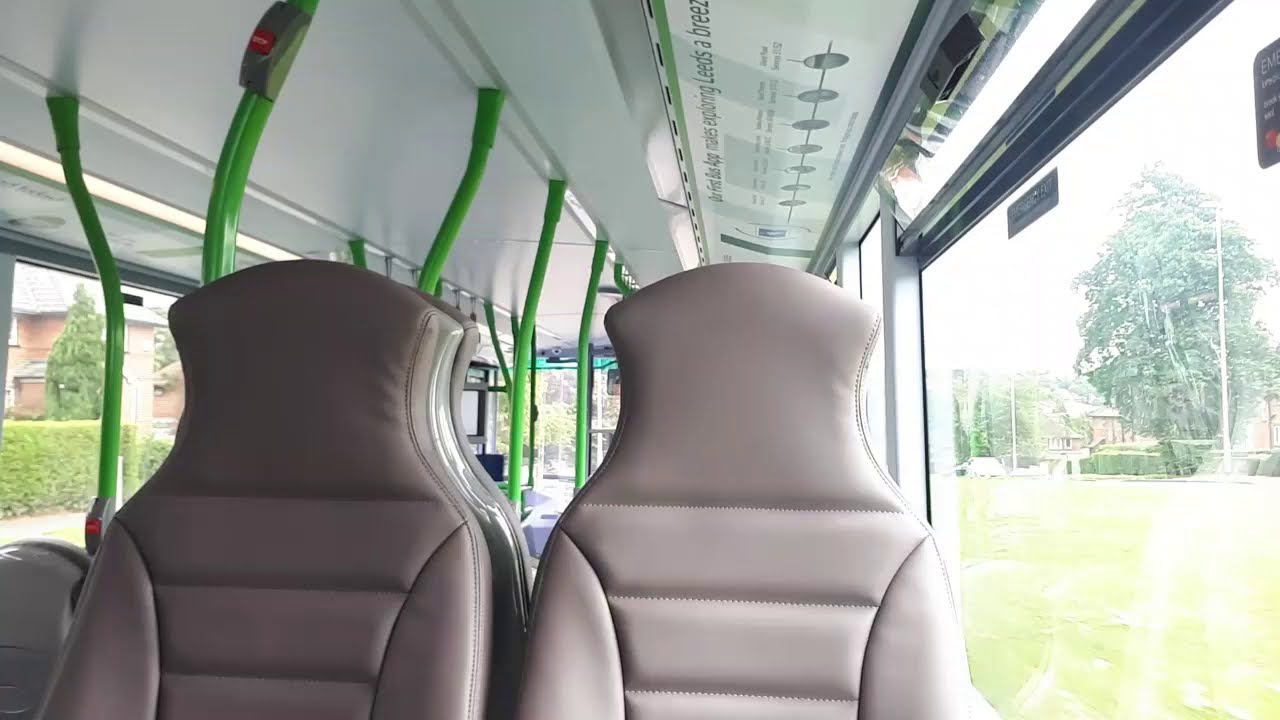This photograph captures the inside of an empty city bus, focused primarily on the center and left section of the vehicle. In the foreground, there are two dark brownish-gray faux leather seats visible from the backrests. Rising from the left side and extending into the background are several green poles, presumably for passengers to hold onto during the ride; these poles are a distinctive grass green color.

On the right side of the image, there is a large window through which the sunny, residential area outside is visible. The view includes a well-trimmed hedge, a stretch of grass, a tall tree that appears to be an oak, and hints of buildings with red walls. Above and positioned in the center near the ceiling, there is an advertisement that reads "Makes exploring Leeds a breeze."

The scene includes various colors such as brown, gray, green, silver, red, and blue, providing a vivid and detailed perspective of a midday bus setting, captured from the viewpoint of someone standing or sitting within the bus.